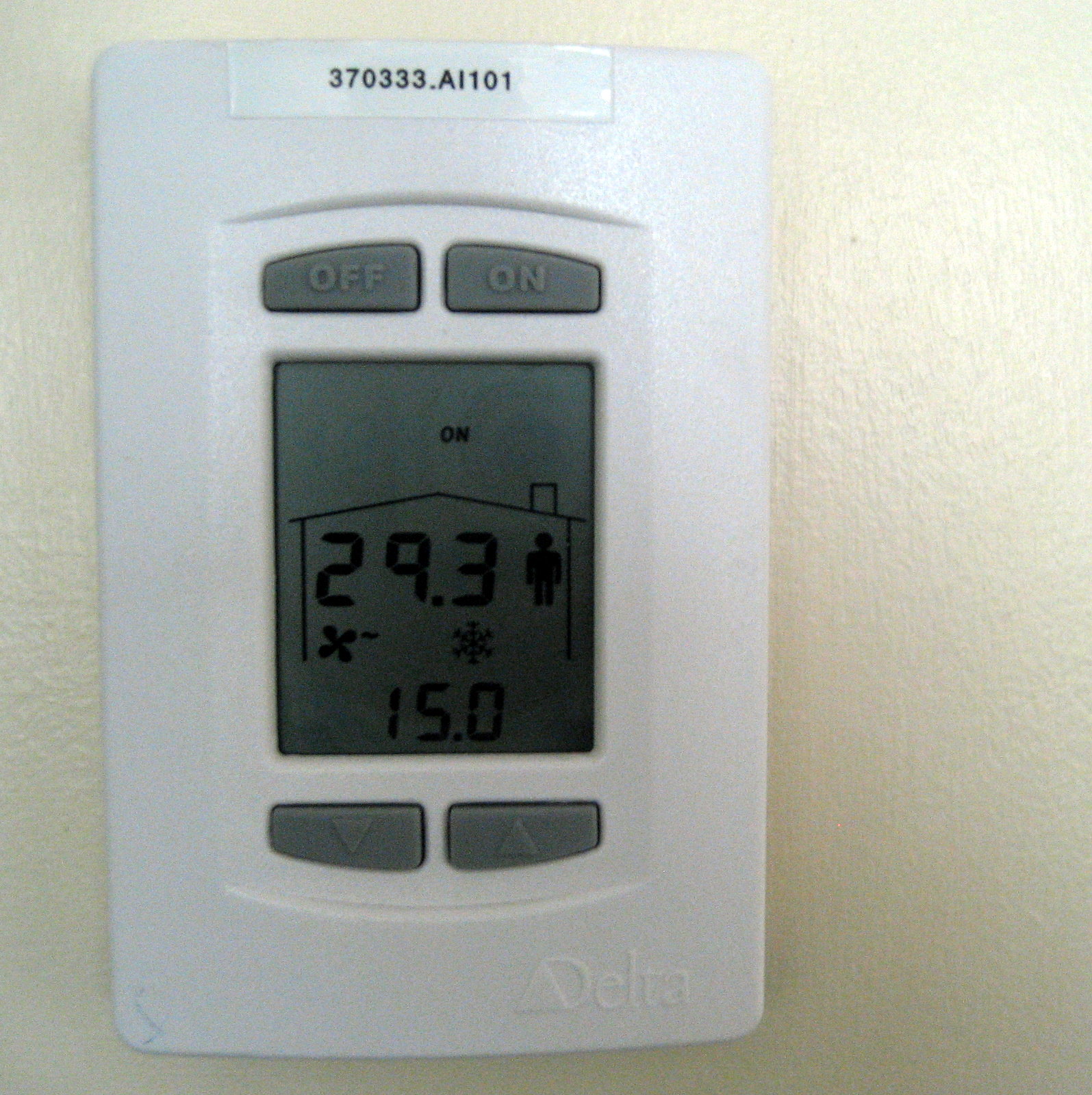A detailed photograph displays an indoor thermostat mounted on an off-white wall with a slight yellow hue. The wall's surface appears reflective. The thermostat, a vertically oriented white rectangular plastic device, is positioned slightly off-center within the image. At its base, there is a raised indentation with the brand name "Delta" subtly embossed on it. A small blue pen mark can be seen in the bottom left corner of the device.

At the top of the thermostat, black alphanumeric labeling on white tape reads "370333.AL101." Below this, an indentation houses two buttons: one labeled "off" on the left and one labeled "on" on the right. The digital readout on the thermostat is marked "on" and includes the outline of a house with a person standing inside. The display shows a temperature of "29.3", a fan icon with a single line indicator, a snowflake symbol, and another temperature reading of "15.0." Beneath the digital readout, there are two buttons for adjusting the settings, one to increase and one to decrease the temperature.

Overall, the image captures the detailed aspects and various elements of the thermostat within the context of its surrounding environment.